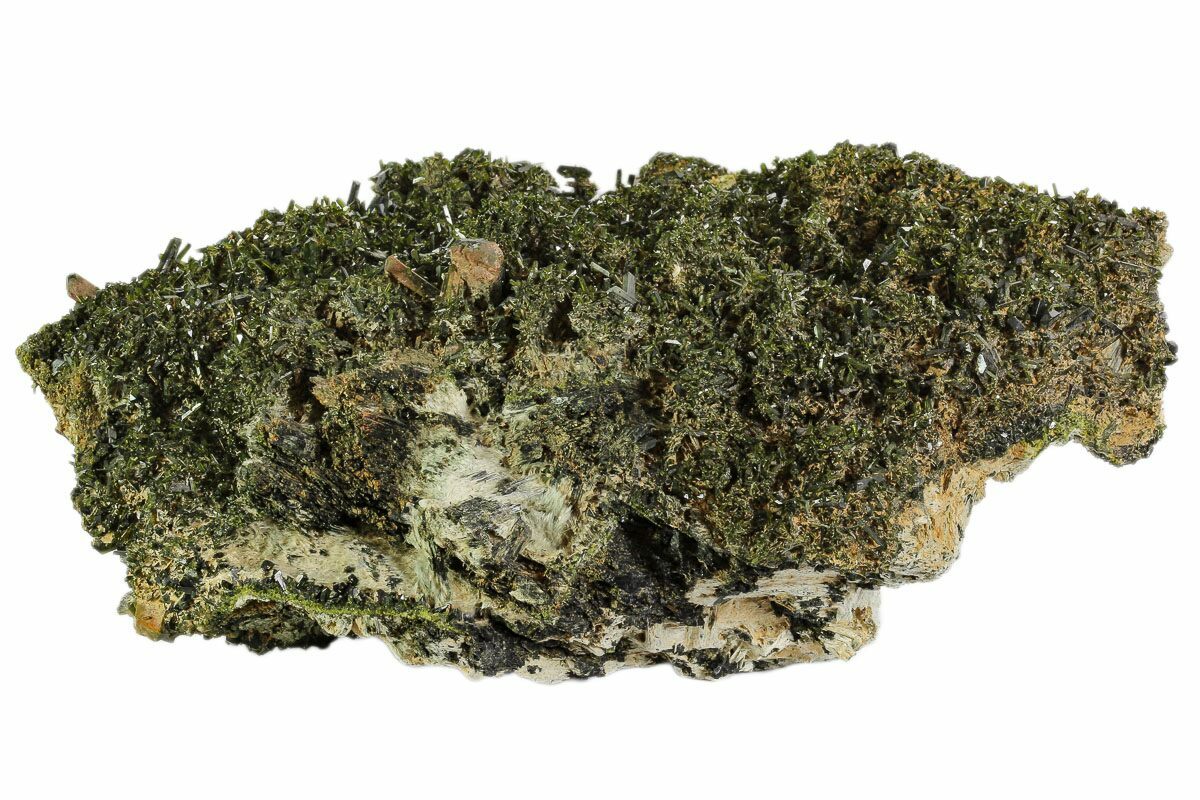The image features a close-up shot of a large rock formation, meticulously isolated against a white background. The object, evocative of either driftwood or an island, is predominantly covered with lush green moss, interspersed with patches of browns, light grays, and light browns. This rugged, irregular piece could easily be mistaken for an aerial view of a tiny, moss-laden island with a shoreline. A notable empty or sandy spot lies in the middle of the formation, adding to its intricate detail. The surface texture and coloration evoke the look of dried seaweed or tree moss. The overall impression is that of a meticulously preserved artifact, possibly even fossilized in some areas, reminiscent of something one might encounter in a museum exhibit.